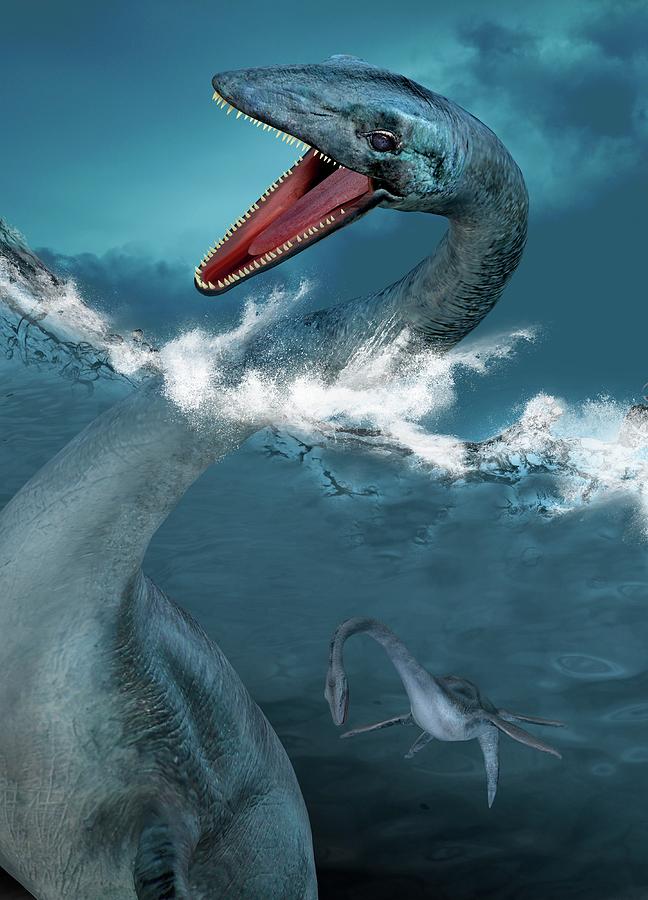This detailed painting, likely digital art, captures a dramatic scene of two Loch Ness monster-like creatures in turbulent waters. The center of attention is an enormous, serpentine beast emerging from the ocean, its open mouth revealing jagged white teeth and a long, red tongue. Its dark eyes are piercing, and its blue skin, marked with wrinkles and possible scars, transitions to white on the chest. Around the creature, white sprays of water splash up, emphasizing its sudden rise from the depths.

The creature's body extends into the water, where multiple fins, resembling oversized oars, are visible, hinting at how it propels itself. To the right, a smaller creature, likely a juvenile of the same species, mirrors the larger one's reptilian features. It has a long neck and multiple fins, with legs and a hump discernible beneath the water's surface. The sky above is filled with dark, shadowed clouds, enhancing the moody and mysterious atmosphere of this Loch Ness-inspired tableau.